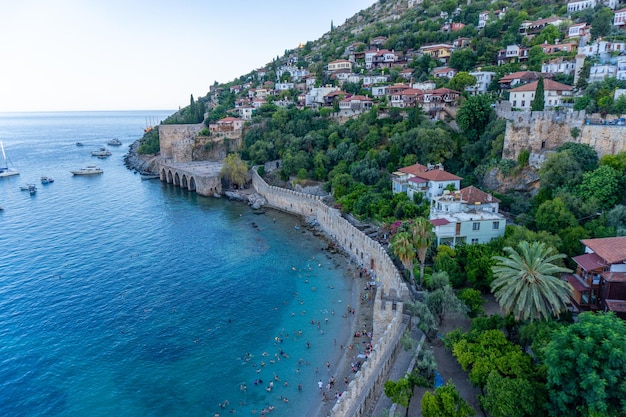This picturesque Mediterranean coastline captures a vivid scene. Dominated by a steep, 45-degree hillside densely packed with about a hundred houses, the land is a patchwork of green trees and residential structures. At the bottom of the slope lies a modest beach, heavily outshone by a large seawall and crowded with beachgoers enjoying the sun and sea. The clear, calm blue waters are dotted with several anchored boats, including a noticeable sailboat on the left side of the image. The upper left corner reveals a serene expanse of blue sky, adding to the tranquil atmosphere. A closer look at the seawall hints at some kind of drainage system, further adding to the intricate details of this coastal landscape.